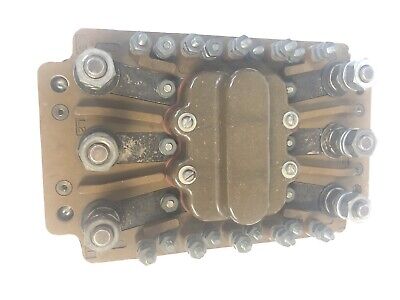The image depicts a rectangular metallic contraption against a white background, characterized by an abundance of nuts and bolts. The device itself has a light tan, almost coppery hue, interspersed with dark black strips of metal. At each corner of the rectangle, there are prominent silver nuts and bolts. Both the top and bottom edges feature around eight bolts each, while the left and right sides have three bolts each. Additionally, the middle section is slightly elevated, with an oval formation secured by four round screws, two on each side. The contraption seems to be more than merely decorative, suggesting it might be a component of a larger mechanical system, possibly for use in a vehicle or machinery.